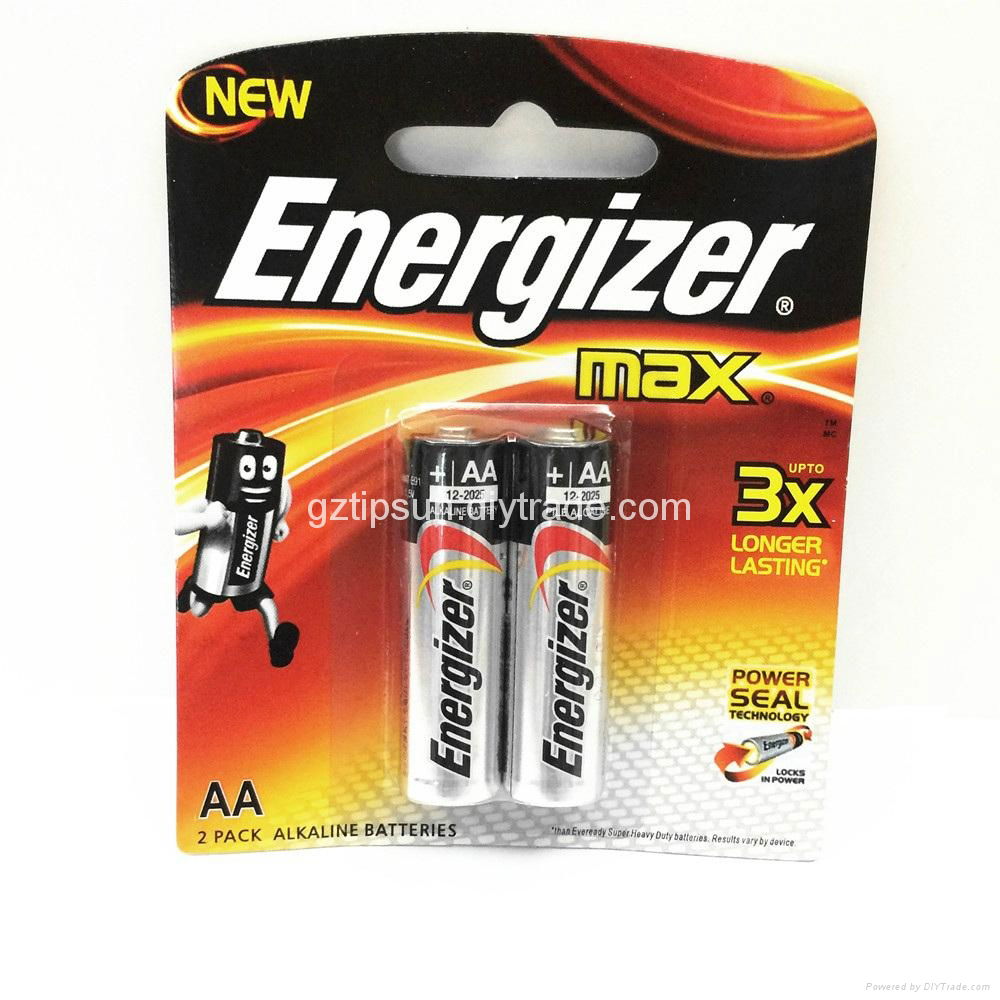This is a highly detailed description of a retail pack of Energizer batteries, captioned meticulously. 

The photograph showcases a pack of Energizer batteries. At the top left corner, a bold yellow label announces "New." The packaging features rounded top and corners and includes a cutout designed for hanging the pack on a display rack. Below this cutout, the word "Energizer" is prominently displayed in large, white letters against a black background. To the right of this, the word "Max" is written over a background of yellow, red, and orange stripes designed to evoke a sense of energy or power.

Midway down the packaging, housed in a clear plastic blister pack, are two AA Energizer batteries. On the left side of the batteries, there's a small character designed to look like a battery with arms, legs, eyes, and a mouth, appearing to be in motion, adding a playful element to the design.

To the right of the batteries, a label states, "Up to 3X Longer Lasting." Further down, another label reads "PowerSeal Technology," accompanied by a graphic of a battery with arrows extending from both the positive and negative terminals, illustrating the feature "Locks in Power."

At the bottom left, the label clearly states "AA," followed by "2 Pack Alkaline Batteries." Finally, in very small print at the bottom right, the text notes, "Heavy Duty Batteries" and "Results vary by device," though the first few words on the left side of this small print are indistinct.